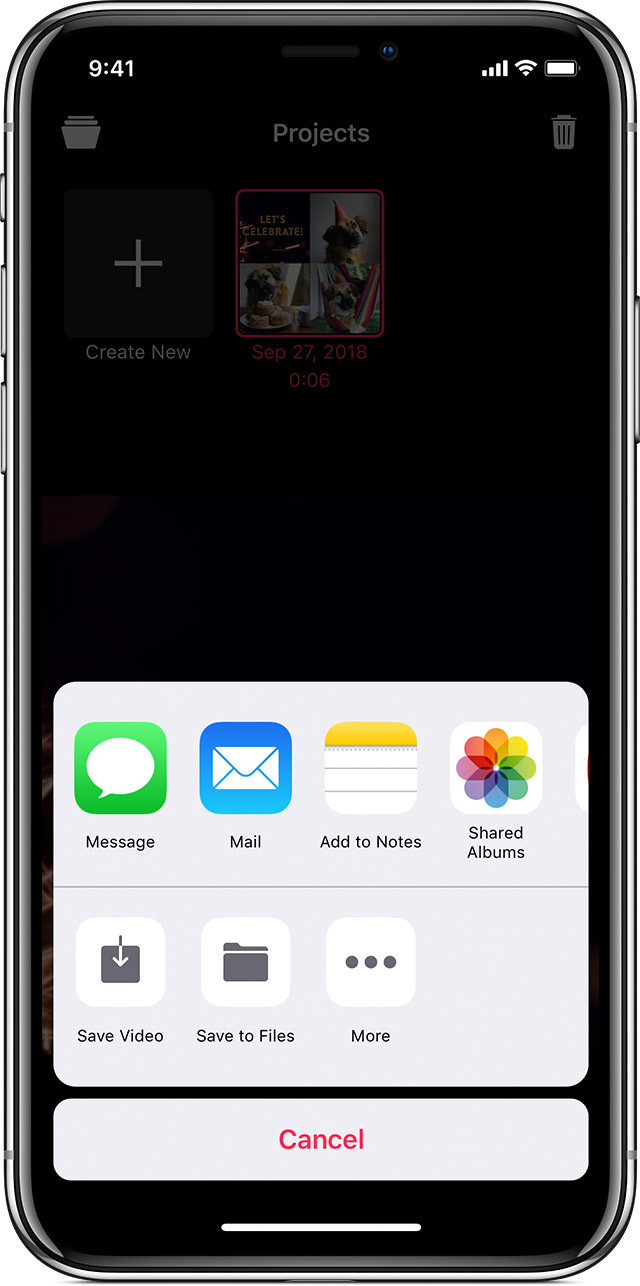This detailed caption describes an image of a screenshot taken on an iPhone. The iPhone, encased in a sleek silver casing, features several key buttons and indicators. On the left side of the device, we see the mute switch and the volume up and down buttons. The right side houses the power button.

In the upper section of the screenshot, the time is displayed on the top left corner, showing 9:41 AM. The cell signal, Wi-Fi, and battery icons are located in the upper right corner. Additionally, the camera unit is visible at the top center of the device.

The main screen background shows the iMovie app. At the top center, we see "US Projects" written prominently, flanked by a trash icon on the right and a tiles icon on the left. There is also a button available for creating a new folder or project. Below this, a project is listed, indicating that it was started on September 27, 2018, and has a duration of six seconds.

At the bottom of the screen, a pop-up tab provides various sharing options, including Message, Mail, Add to Notes, Shared Albums, Save Video, Save to Files, and More. There is also an option to cancel the sharing process.